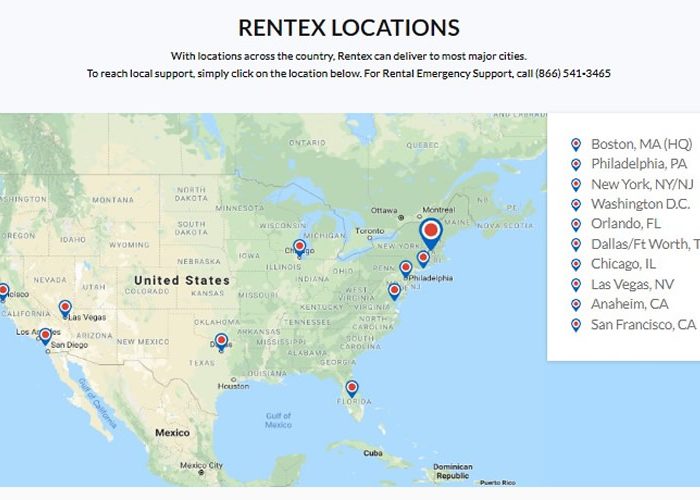Rintex offers extensive delivery services to most major cities across the country. For emergency support, you can click on the corresponding location below to initiate a support call. Please contact 1-866-541-23465 for assistance in the following locations: Boston, MA; Philadelphia, PA; New York, NY; Washington, DC; Orlando, FL; Dallas, TX; Fort Worth, TX; Cocoa, IL; Las Vegas, NV; Hannah, CA; various locations in Maine; Philadelphia (repeated); Toronto, ON; various locations in Tennessee; various locations in Kansas; Mexico; multiple regions in California; and the Gulf of Mexico.